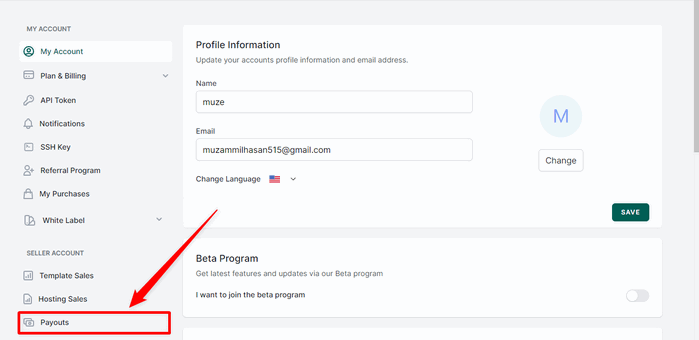This detailed caption describes the layout and features of an account information page:

---

The screenshot displays an account information page with a light grey background. On the left side, a vertical menu lists various options such as "My Account," "Plan and Billing," "API Token," "Notification," "SSH Key," "Referral Program," "My Purchases," and "White Label." Below these, under the "Seller Account" section, the options "Template Sales," "Hosting Sales," and "Payout" are visible. The "Payout" option is highlighted with a red rectangular border, and a red arrow pointing from the top emphasizes this section.

On the right side of the page, there is a profile information section with a header that reads, "Update Your Account Profile Information and Email Address." The displayed profile information includes the name "Muse" and the email address "musemilhasan518@gmail.com." There is an option to change the language, and a "Change" link on the right side for modifying profile details. Below this, a green "Save" button is present, which is used to save any changes made to the profile information.

At the bottom of the profile section, there is an invitation to join the beta program with the text, "Get the latest features and updates via our Beta Program." Adjacent to this message, there is a slider button that is currently turned off.